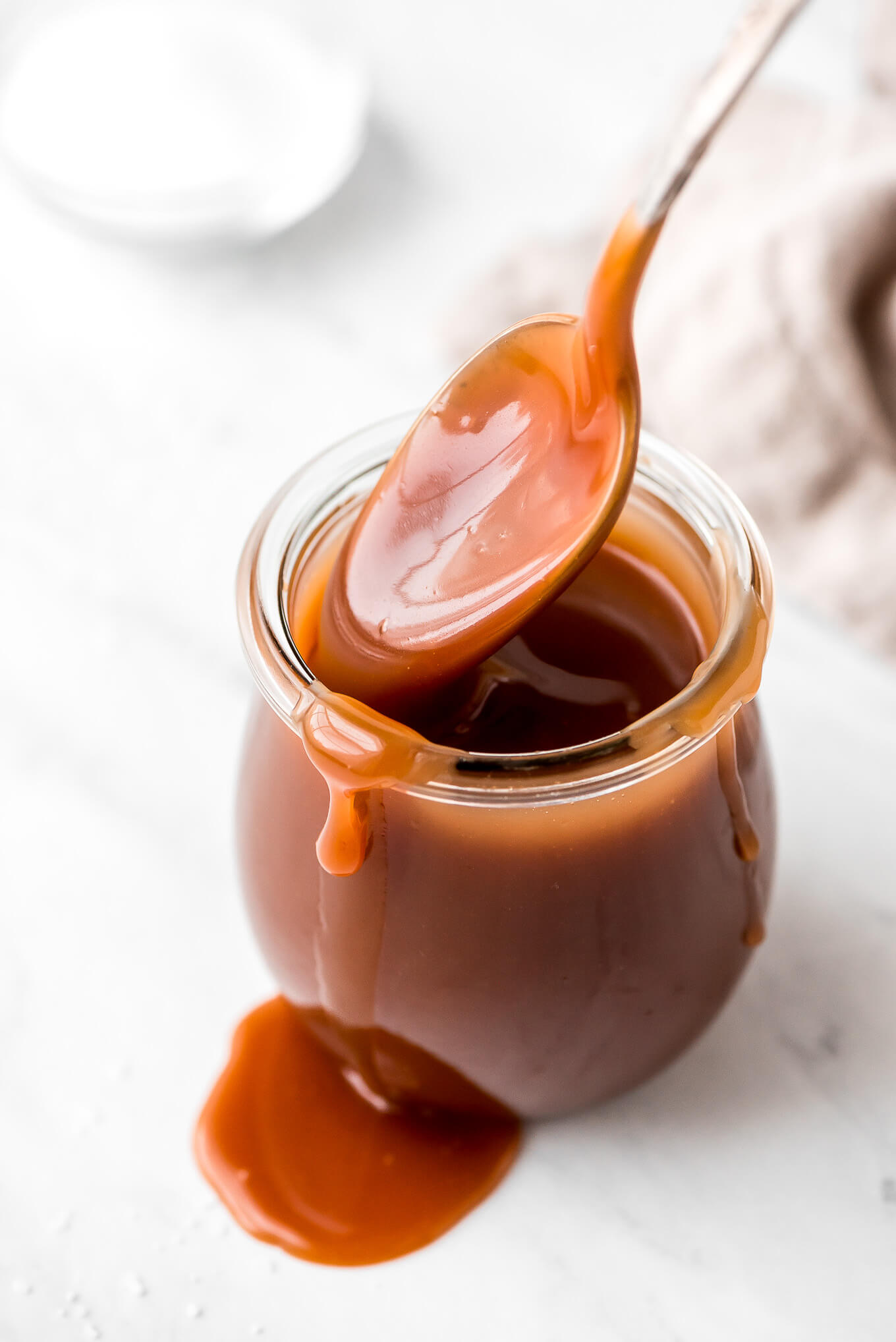In the foreground of the image, a small, rounded crystal jar sits on a white marble counter, filled to the brim with a thick, gooey caramel sauce. The caramel is visibly dripping down both the front left and the right side of the jar, forming a little puddle on the counter beneath the front of the jar. A silver spoon, coated with caramel that reaches halfway up its handle, stands upright in the jar. The indentation in the caramel around the spoon suggests it has just been stirred. In the blurred background, there's a white dish and possibly a cloth on the counter, contributing to the kitchen setting. The close-up shot captures the lusciousness of the caramel, making it an enticing image suitable for a kitchen decor.